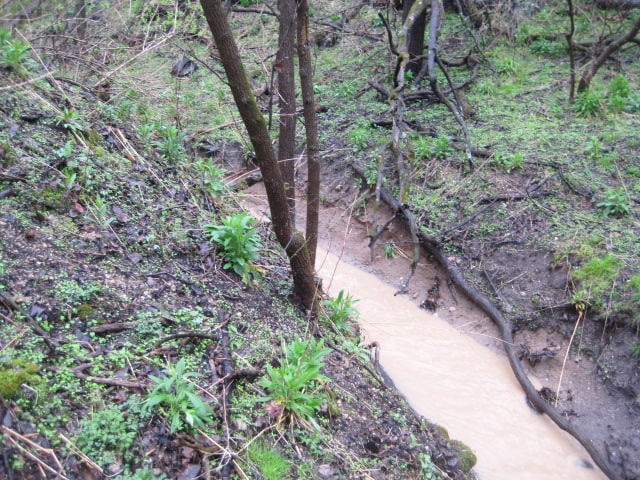This landscape-oriented color photograph captures a natural forest setting, focusing on a muddy creek coursing through the scene. The creek, beginning in the bottom right corner of the image, winds its way toward the center before disappearing around a hill. The stream's light brown, muddy water is flanked by wet, brown dirt banks that slope upwards to the left and right. 

In the center of the image, on the left bank, stands a large tree with multiple trunks surrounded by spotty green plants and fallen twigs. Both sides of the creek are adorned with a mix of fallen branches, twigs, and patches of green grass. The right bank features a single limb that runs alongside the creek. The surrounding forest is characterized by a variety of thin tree trunks and dense underbrush, contributing to the image's rich, earthy tones of brown, tan, green, and occasional shades of black. The photograph exemplifies representational realism, capturing the serene yet rugged beauty of this woodland area.